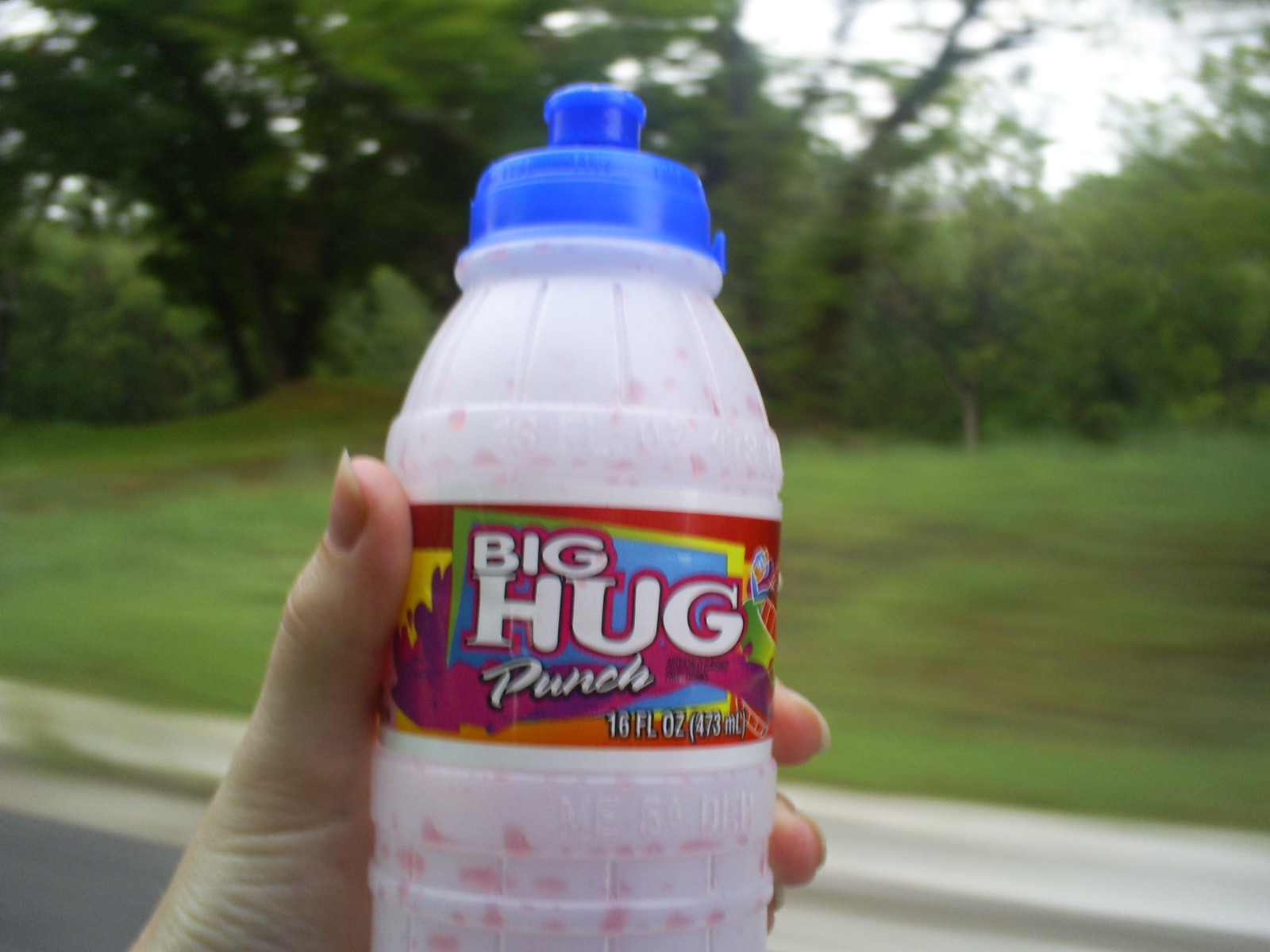A person is holding a bottle labeled "Big Hug Punch" in white letters. The label details that the product contains 16 FLOZ (473 ML). The design features a vibrant red background with a central blue square bordered in yellow, accented by dynamic red splashes. The bottle itself is made of clear, slightly milky plastic, adorned with red droplets on the inside. The lid is blue and round, equipped with a small, narrow blue spout at the top. In the backdrop, there is a lush, green landscape with grass and trees, accompanied by a gray sidewalk adjacent to a paved road.